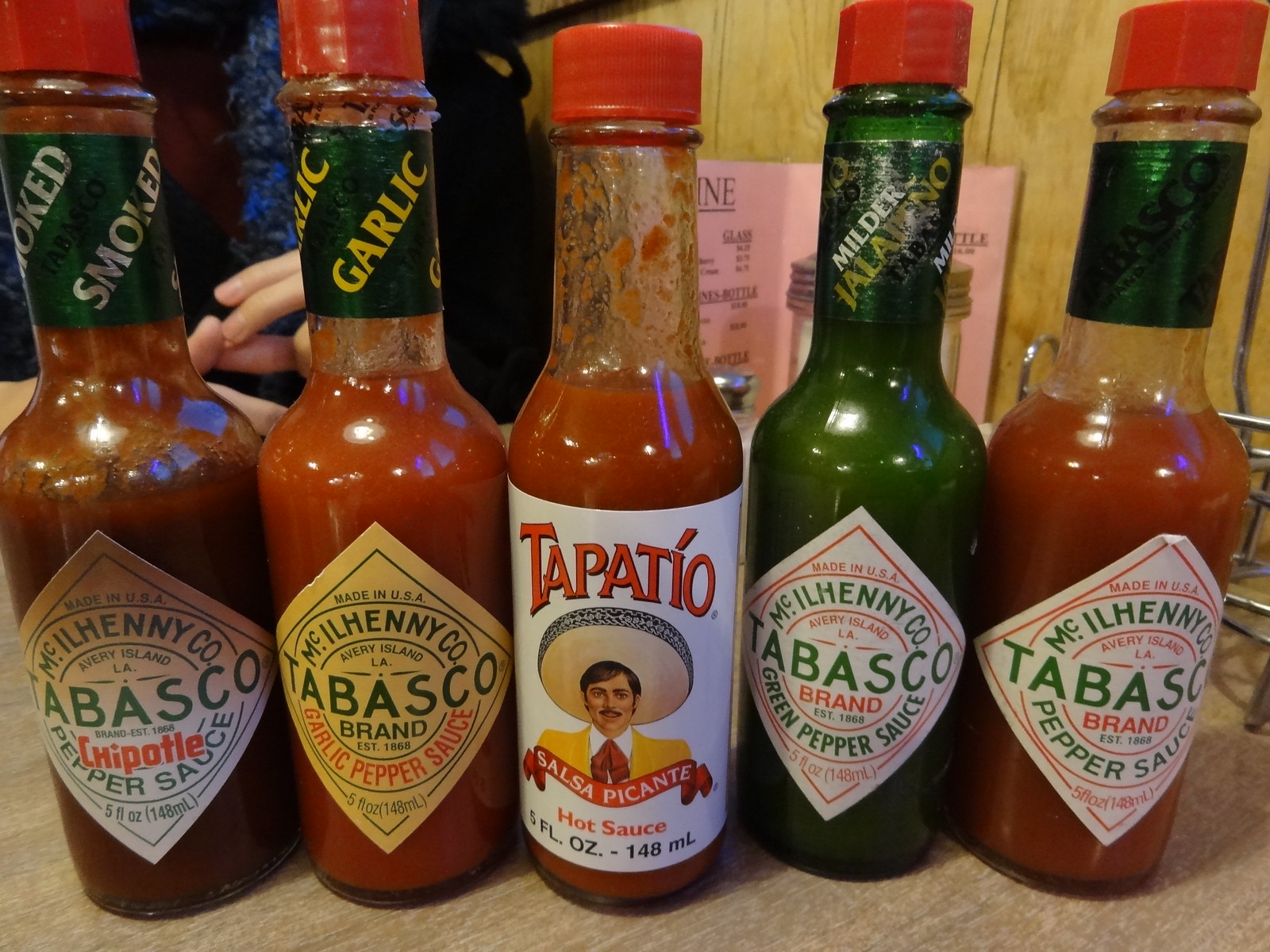The photograph, taken indoors at a restaurant, showcases a wooden table adorned with five different bottles of hot sauce. The backdrop features nostalgic wood paneling from the 70s, with pink menus propped against it. Across the table, a light-complexioned hand is partially visible, possibly belonging to a seated diner. 

On the table, from left to right, the lineup begins with a bottle of McIlhenny Company Tabasco Chipotle Pepper Sauce, recognized by its "smoked" band around the neck. Next is the Tabasco Brand Garlic Pepper Sauce, featuring a "garlic" band. In the center is a bottle of Tapatio Salsa Picante Hot Sauce, distinct for its label depicting a man in a yellow suit, red tie, white collar, and sombrero. Following that, there's the Tabasco Brand Green Pepper Sauce, marked as "Milder Jalapeno" with a green hue. The final bottle is the classic Tabasco Brand Pepper Sauce, noted for its fiery red color.

All Tabasco bottles sport their iconic red caps, aligning harmoniously with the traditional shape and branding. The Tapatio bottle stands out with its unique image and yellow label, differentiating it clearly from the others. This carefully arranged selection of hot sauces, along with the restaurant setting, evokes a quaint, vintage dining experience.